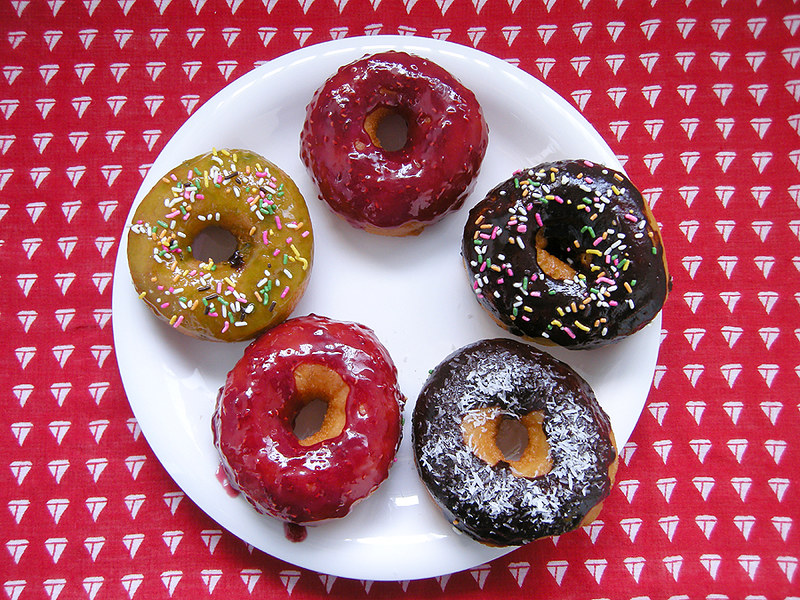This is a detailed photograph taken from an overhead perspective of a white plate containing five doughnuts, positioned on a red tablecloth adorned with white diamond patterns featuring red T-shaped separations. Centered on the plate is a vibrant assortment of doughnuts, each with distinct toppings. At the 12 o'clock position, there's a doughnut with bright red glaze. Moving clockwise to 3 o'clock, a chocolate-frosted doughnut is decorated with multicolored sprinkles in green, white, and yellow hues. At the 5 o'clock spot, another doughnut with rich chocolate icing is topped with coconut shavings. Continuing around to 7 o'clock, a second red-glazed doughnut is situated. Finally, at approximately 10 o'clock, there's a tan doughnut with yellow icing and scattered with blue, white, and yellow sprinkles. The entire setting exudes a vibrant and appetizing visual appeal against the bold and patterned backdrop.